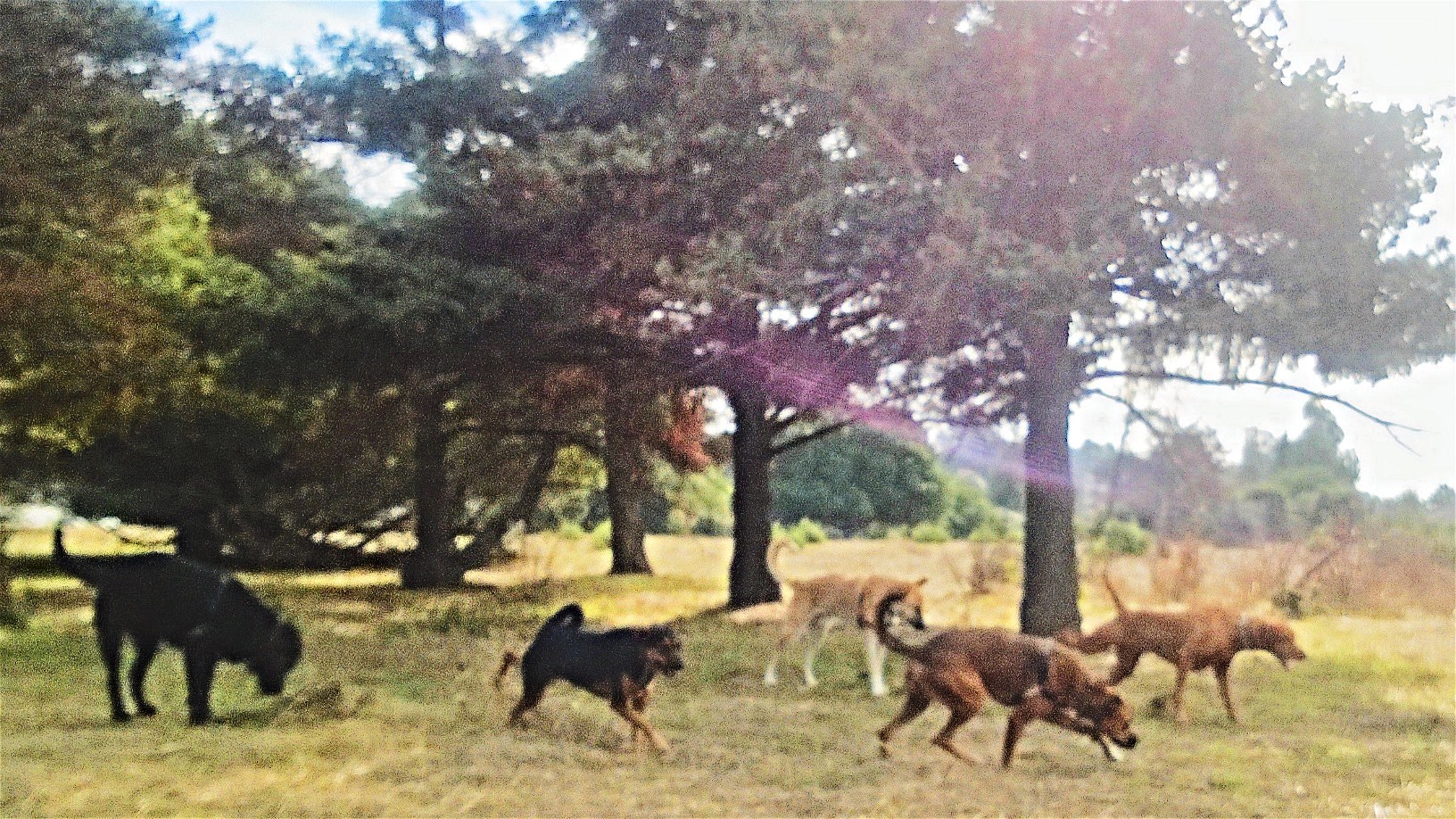This is a grainy and blurry, high-contrast photograph, seemingly cropped from a larger picture, depicting a group of five dogs in motion across a slightly browned, green field, likely taken during the summer. The focal point of the image is the five dogs, each with distinct markings and colors. To the left is a large black dog, followed by a black dog with brownish feet, possibly a shepherd with a curled tail. Next, a light brown dog with black facial features and white legs appears to be sniffing the ground while moving. Behind them, there are two more dogs: one with a reddish-brown smooth coat and another lighter brown dog, both seem to be running. In the background, towering evergreen trees and mature deciduous trees are set against a backdrop of lush but blurry greenery, with beams of sunlight filtering through. The dogs are all moving to the right, possibly reacting to something or someone approaching.